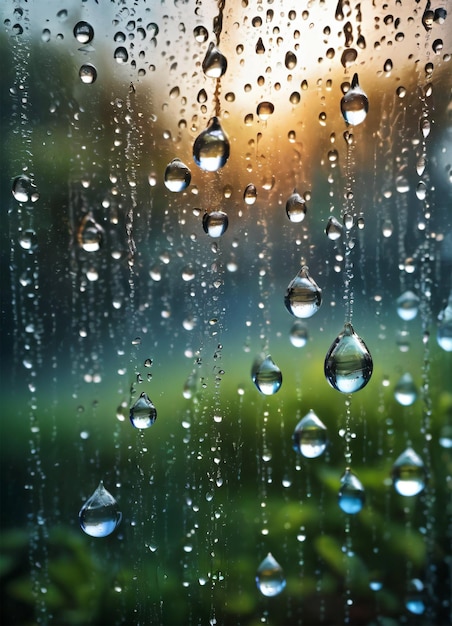This image captures a rectangular photograph in portrait orientation, showing a window covered with water droplets from a rainstorm. The glass pane has water droplets on both its interior and exterior, with larger droplets at the top middle and bottom right; each droplet is teardrop-shaped, more rounded at the bottom than the top, with multiple smaller droplets being left behind by the larger ones as they slide down. The backdrop through the window is blurred, revealing indistinct colors of orange, blue, green, and white, suggesting a landscape with a green yard and trees below, a stretch of blue perhaps indicating the sky or distant horizon, and touches of orange and yellow hinting at a sunset or sunlight peeking through the dark gray clouds. The overall composition is dominated by the interplay of the water droplets on the clear glass and the softly blurred, colorful background.